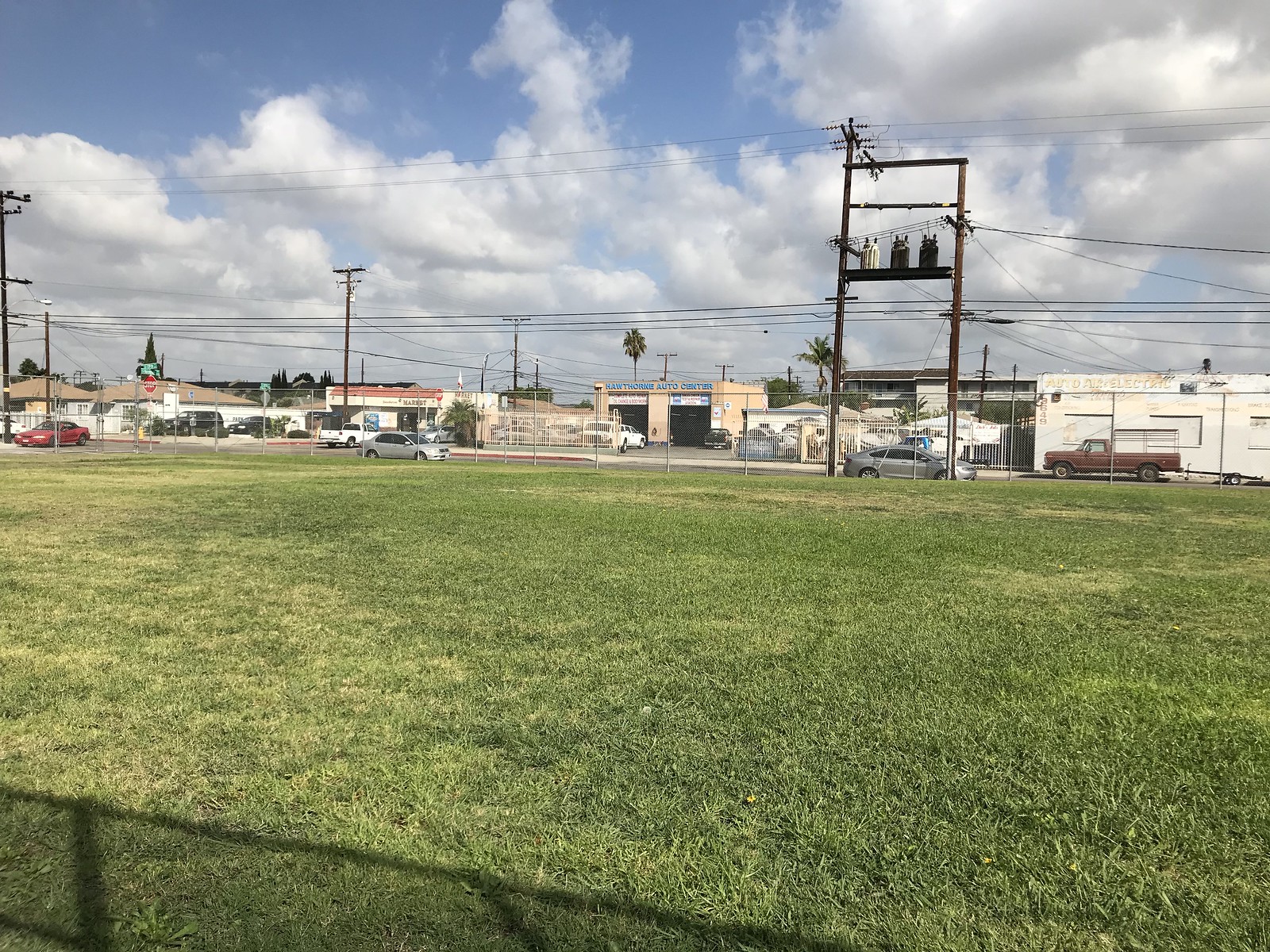This photograph captures an expansive field stretching towards a cluster of buildings and power lines on the horizon. The horizon line divides the image horizontally at the midpoint, juxtaposing the verdant grass against the blue sky. In the bottom left corner, the shadow of a fence slants diagonally from left to right, with the pole shadows casting a darker impression compared to the lighter shadows of the netting. The grass in the field looks freshly mowed, though some patches display a slightly yellowed, dying hue, contrasting with the otherwise healthy green expanse.

Beyond the grassy field lies a busy road with vehicles traveling in both directions. Dominating the right third of the photograph is a large wooden power line structure. Behind the vehicles and power lines, various buildings come into view. The building on the far right boasts prominent graffiti lettering, while the other structures are predominantly single-story and appear to have fenced yards, suggesting they could be car dealerships or garages. As the line of buildings extends to the left, they seem more residential in nature.

Multiple power lines run horizontally across the image, also veering off at an angle down a side road. The sky overhead is a vibrant blue, scattered with abundant white clouds. The clouds exhibit grey undersides while their tops remain white and wispy, adding texture to the sky.